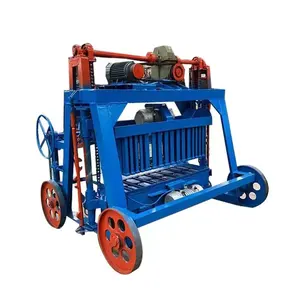The image presents a detailed photograph of an old-fashioned mechanical device predominantly made of metal. The contraption features a sturdy, bright blue frame adorned with vertical bars arranged in close rows, giving the impression of a metal picket fence. Central to the machine are four wheels: two visible on the left side, painted red with six holes each, and another visible at the top right, painted blue. The fourth wheel is obscured from view. At the top of the device sits a complex assembly resembling an engine, composed of black and gray components accented with red trim. Intersecting the machine horizontally is a red metal bar flanked by two black cylinders with red ends. A notable feature is a circular blue hand crank situated above the red wheels, suggesting a manual operation function. The entire assembly is set against a stark, white background, highlighting the vivid colors and intricate details of this metallic apparatus.